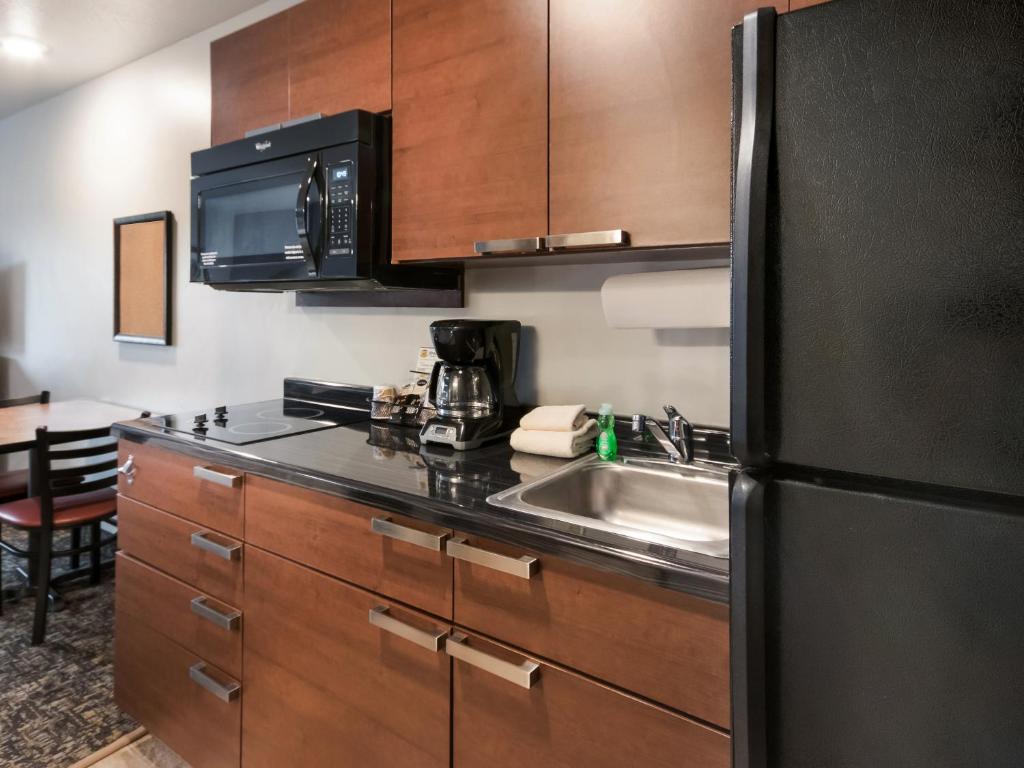This photograph depicts what appears to be a workplace kitchen or breakroom. The right side of the image showcases a black refrigerator adjacent to a sink, which is embedded within a large counter space that features multiple chocolate brown cabinets and drawers beneath it. Above the sink, a paper towel roll is suspended, likely mounted to the wall. The counter area is also home to a black coffee machine and dish soap, with hand towels nearby. Just above, a black microwave is mounted to the wall, and a brown cupboard hangs above it. Below the microwave, the countertop is largely empty, except for a few small items. On the left side of the image, a small table and chair set can be seen, giving the room a breakroom feel. The walls are gray, accentuated by a black and brown empty frame matching the room's color scheme. Additionally, a built-in electric range is noted, and the floor features a woven gray-brown rug. The overall aesthetic combines stainless steel appliances with a consistent dark brown and black color palette.